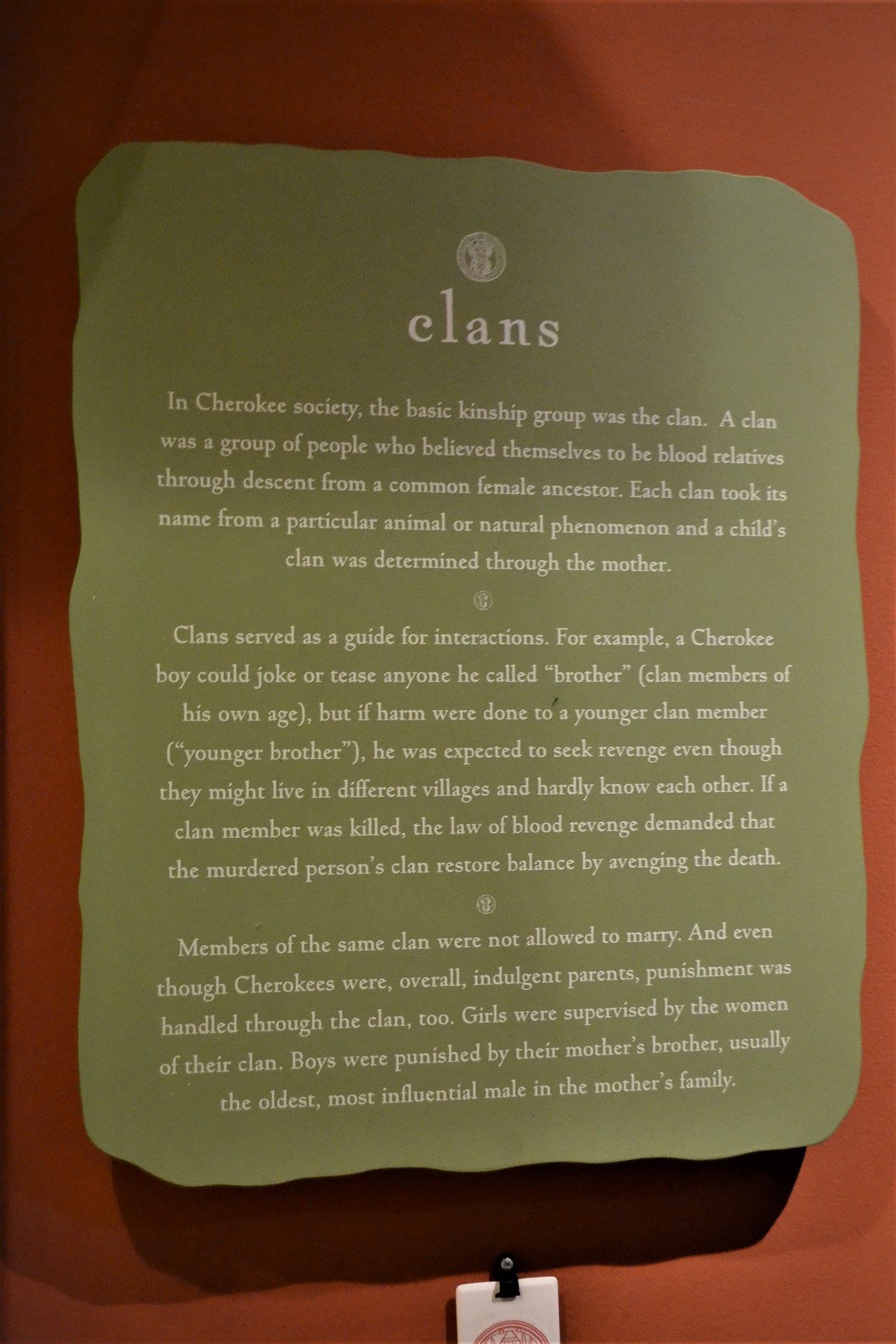The image showcases a light green plaque set against a light brown background. The plaque is rectangular with curved sides and includes a small tab hanging below, possibly attached by a black clip. At the top, there is a small circular logo or icon, followed by the title "Clans" in white print. The main body of the plaque features three paragraphs in fine print. The text elaborates on the role of clans in Cherokee society, explaining that a clan was a kinship group where members considered themselves blood relatives through descent from a common female ancestor. Each clan derived its name from an animal or natural phenomenon, and membership was matrilineal, determined through the mother. Clans dictated social interactions, prohibiting intra-clan marriages, and handling discipline within the group. Girls were supervised by the women of their clan, whereas boys were disciplined by their mother's brother, typically the eldest and most influential male in the family. The document also notes the cultural practices of joking or teasing among clan 'brothers,' and the law of blood revenge that required avenging a clan member's death to restore balance. Shadows cast beneath the plaque on the background add a subtle depth to the scene.